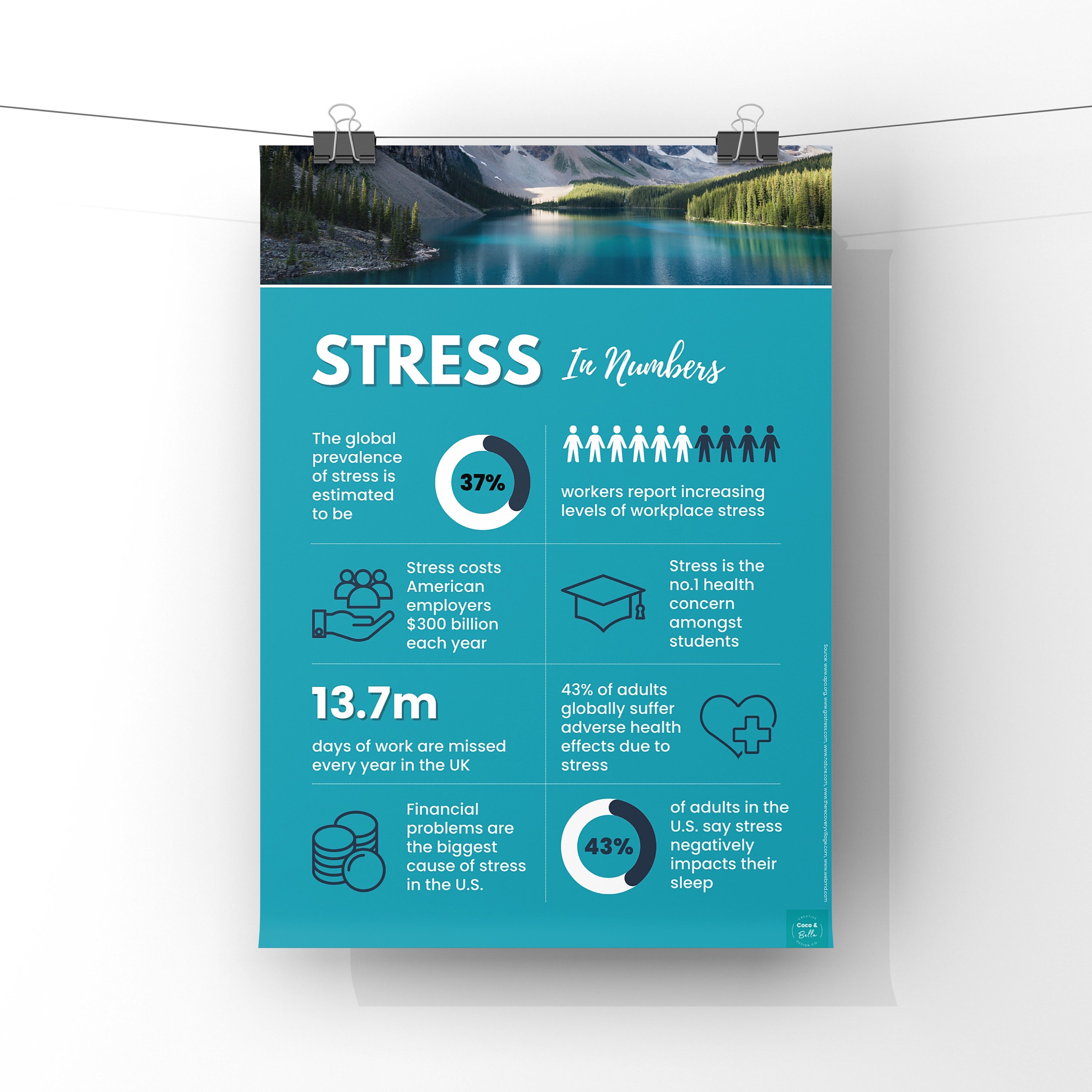The image is of a flyer titled "Stress in Numbers," held up by two black binder clips, one at each top corner, attaching it to a piece of wire. The top quarter of the flyer features a serene outdoor scene of a blue lake with snow-capped mountains and green trees meant to convey tranquility. The rest of the flyer is a light blue or aqua background with black and white text detailing various statistics on stress. Key points include: the global prevalence of stress at 37%, stress costing American employers $300 billion annually, 13.7 million workdays lost each year in the UK due to stress, and financial problems being the leading cause of stress in the US. It also notes that 43% of adults in the US report stress negatively impacting their sleep, 43% of adults globally experience adverse health effects due to stress, and stress is the top health concern among students. Additionally, most workers indicate rising levels of workplace stress. The flyer uses visual markers such as white and black silhouettes to illustrate the impact of stress.